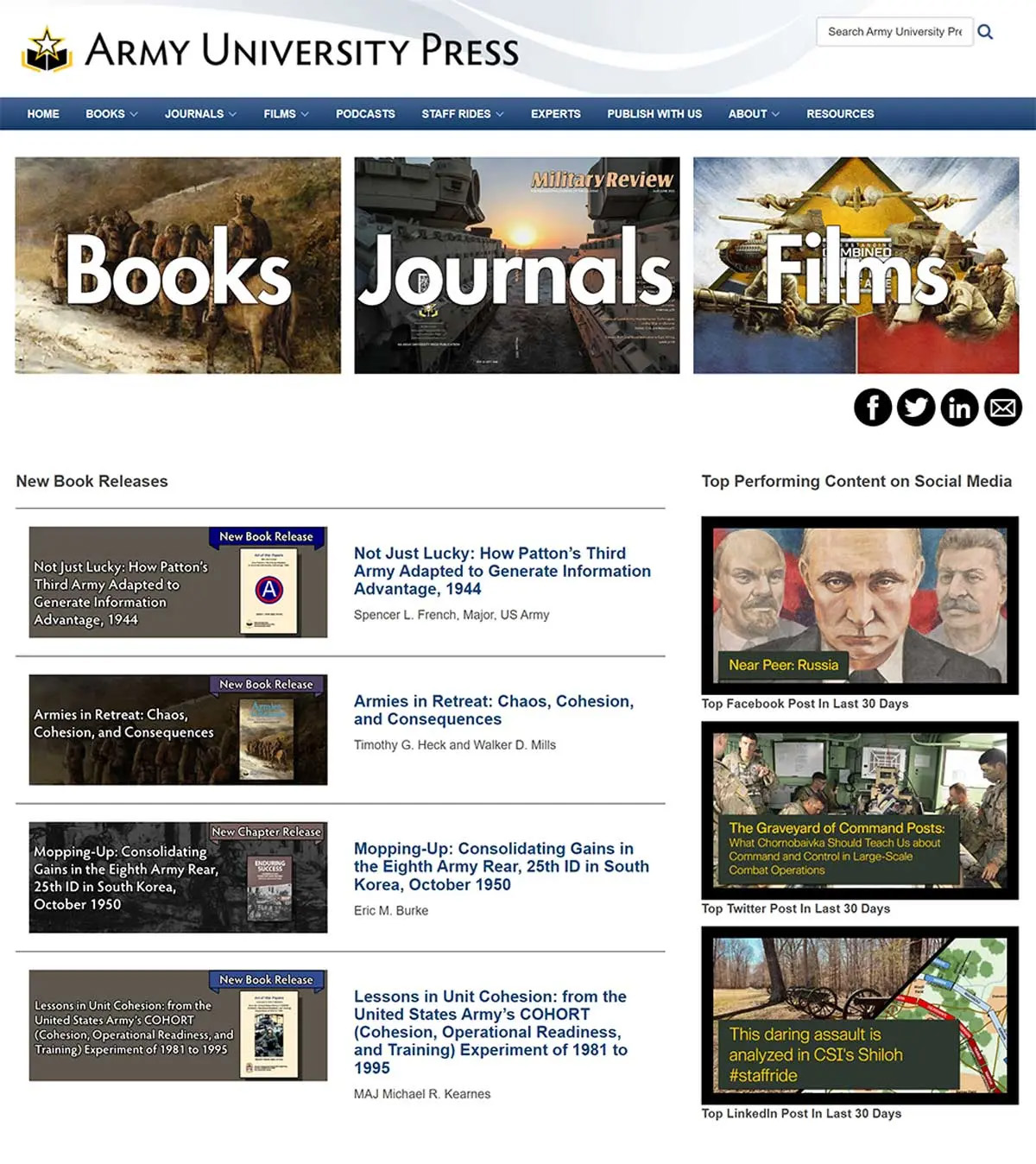At the top left of the image, a gray banner features the text "Army University Press." On the top right, a magnifying glass icon includes a data field with the phrase "search Army University Press." Below this, a blue navigation bar is displayed with white font. The navigation options listed are: Home, Books (with a pull-down menu), Journals (with a pull-down menu), Films (with a pull-down menu), Podcasts, Staff Writes (with a pull-down menu), Experts, Publish with Us, and Resources.

The body of the image contains three prominent photographs, each labeled with large font text: "Books," "Journals," and "Films." Below these images, there is a section for new book releases on the left, showcasing four titles. 

The first book, titled "Not Just Lucky: How Patton's Third Army Adapted to Generate Information Advantage in 1944," is accompanied by a photograph. Below this title is a gray line separator.

The second book title, "Armies in Retreat: Chaos, Cohesion, and Consequences," is also separated by a gray line.

The third book is titled "Mopping Up: Consolidated Gains in the English on the 8th Army Rear, 25th ID in South Korea, October 1950," with another gray line separating this listing from the subsequent content.